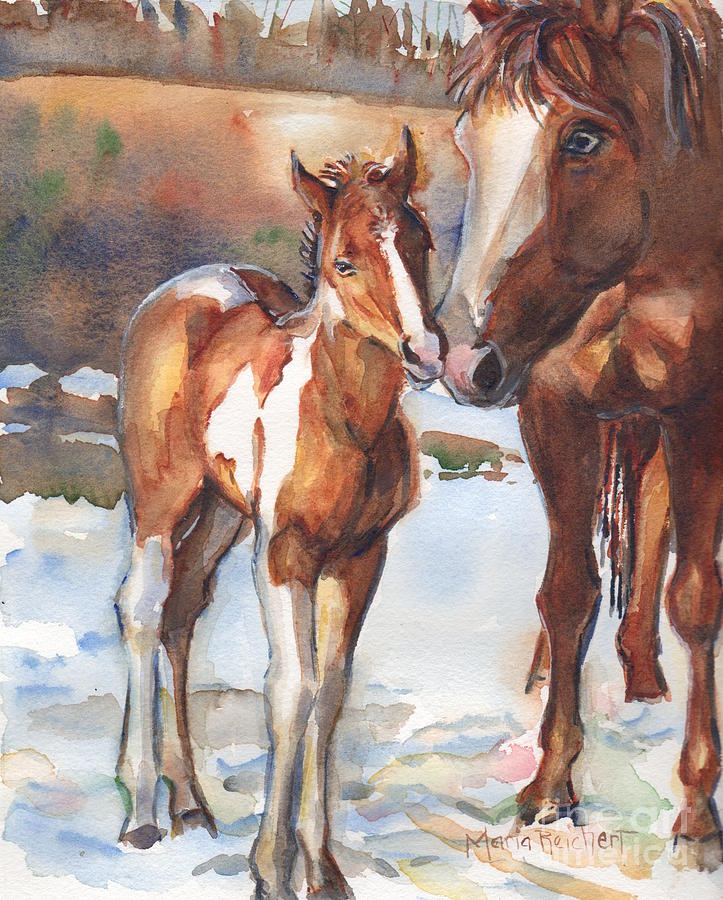This watercolor painting depicts a touching moment between two horses, a larger adult horse and a smaller foal, set against a snowy winter landscape. The painting measures vertically and features the mother horse on the right, standing mostly facing forward with her head slightly turned to showcase the left side of her face. Detailed with a white blaze down her brown face, the mother horse's pink-tinged nose almost touches the foal's nose in a tender gesture. The adult horse's body is visible from ears, neck, and mane through to her chest, legs, and tail. The foal, positioned on the left, is portrayed with an intricate coat of brown and white patches, white legs, and more spots. Both horses stand on a snowy bank, their figures etched in rich watercolor strokes that give the snow textured shadows in hues of gray, yellow, and blue. The background subtly hints at a body of water and a flat field with grasses and trees, all depicted as soft, indistinct smudges of color. Adding a personal touch, the name "Maria Reichert" is painted at the bottom alongside a faint watermark reading "the art," blending into the white snow.